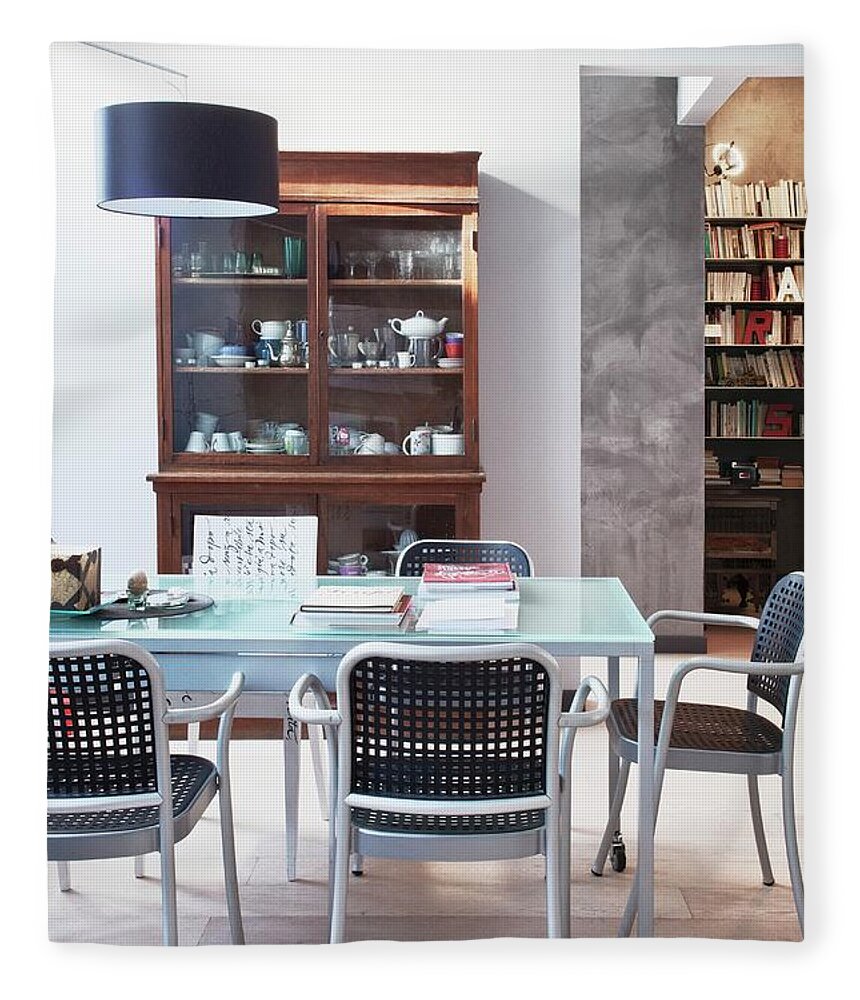The photo captures a dining room with a powder blue glass table, framed in a blue to silver gradient. Surrounding the table are four chairs, each featuring a see-through pattern of small squares on their black backs, with a sleek silver frame. On the table, there are scattered papers and books along with a small tray, possibly holding some indistinguishable items, and an ornate candle with a black and yellow design.

Against the wall, there's a large wooden hutch filled with an assortment of glasses, tea cups, and other tea utensils, mostly in white, clear, and hints of red. The right side of the photo features a brown bookshelf with seven shelves crammed with books and a small cabinet underneath. Hanging above the table is a black circular lamp, adding a focal point to the room, which has a mix of white and brown linoleum tiles on the floor. The walls are predominantly white with a gray accent area, giving the room a subtle contrast. Overall, the eclectic mix of elements suggests a cozy and functional space, potentially serving as a combined dining area and informal library.